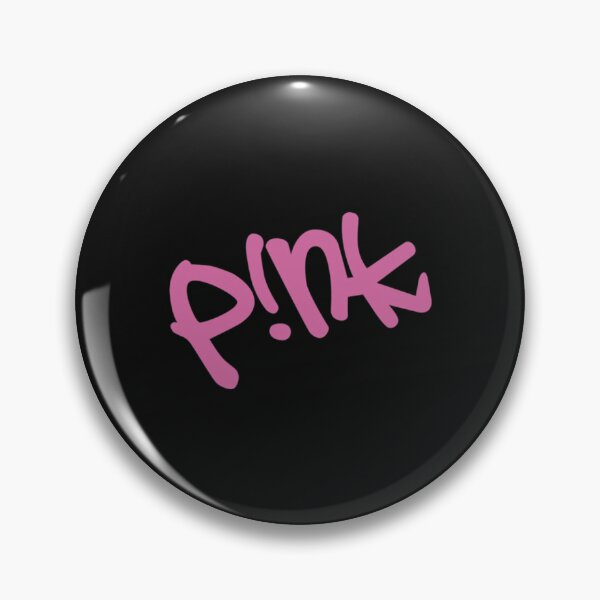The image features a large, round, black pin button set against a plain white background. Dominating the composition, the button's polished, shiny surface reflects light prominently, revealing white highlights that suggest a light source from above. In the center of the button, in lowercase graffiti-style font, the word "pink" is displayed in vibrant pink colors, with the "i" uniquely stylized as an exclamation point. The button, which is suspended in the center with shading visible beneath it, suggests an element of support for a cause or artist, possibly the musician Pink.